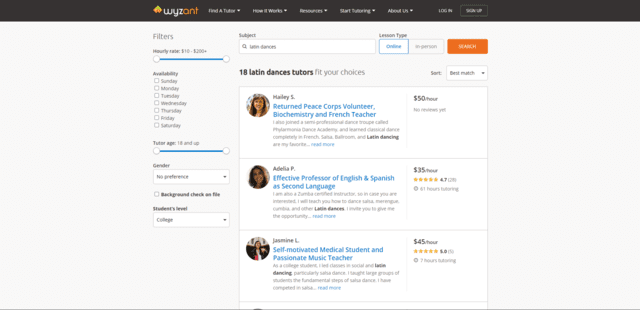The image is a screenshot of search results from the website Wyzant. The search results are for "Latin dance tutors" and show a total of 18 available tutors. The list displays their names, with the first tutor being Hayley S, the second Adelia P, and the third Jasmine L. The names are written in small text, making them slightly difficult to read, but these are the identifiable names in the results.